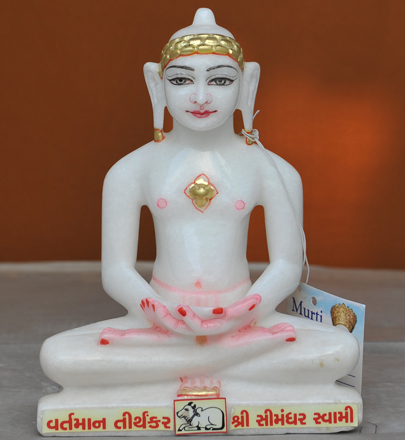The image features a detailed ivory-colored statue, closely resembling a Buddha, seated on a grayish surface with an orange-brown background. The figure is characterized by several notable features: a gold headband, dangling gold earrings, large dark eyes with outlined but colorless pupils, and a slightly smiling red mouth with pronounced lipstick. Its earlobes are elongated, and both have light pink tips. The statue’s nipples, palms, soles of the feet, and groin cloth are all pink. Centered on its chest is a gold flower or diagram. The statue's hands rest in an 'Indian-style' position, with palms facing upwards. Inscribed on the base is a foreign language, which also contains a legible M-U-R-T-I in blue text. Additionally, there is a blue card with a gray image balanced to the right side of the figurine.